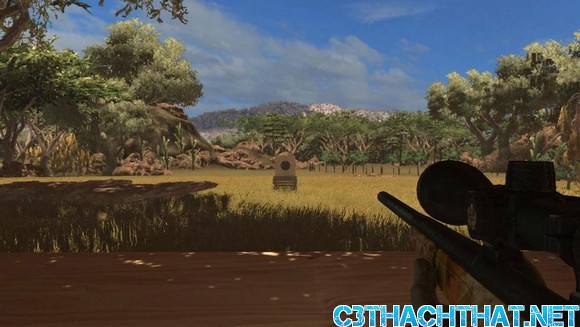The image is a detailed screenshot from a video game that depicts a natural and somewhat wild setting. The scene features a blue sky scattered with white clouds and a distant mountain with a slightly snow-capped peak. The midground showcases a row of tall, green trees interspersed with dry knee-high grass of a brownish hue, indicative of a warm environment. 

In the field, there is a conspicuous target, characterized by a small black dot at its center within a brownish object. Closer to the camera, the vibrant natural setting transitions into a murky river of dark, brownish water, adding to the serene yet rugged ambiance of the scene. 

At the bottom right corner of the image, partially illuminated by light filtering through the treetops, a rifle with a sniper scope is visible, positioned as if being aimed, yet no person is shown. 

Additionally, the text "C3THACHTHAT.NET" appears in blue at the bottom right, contributing to the digital, game-like essence of the image. Overall, the scene combines elements of lush greenery, dry grasslands, and aquatic features under a clear sky.